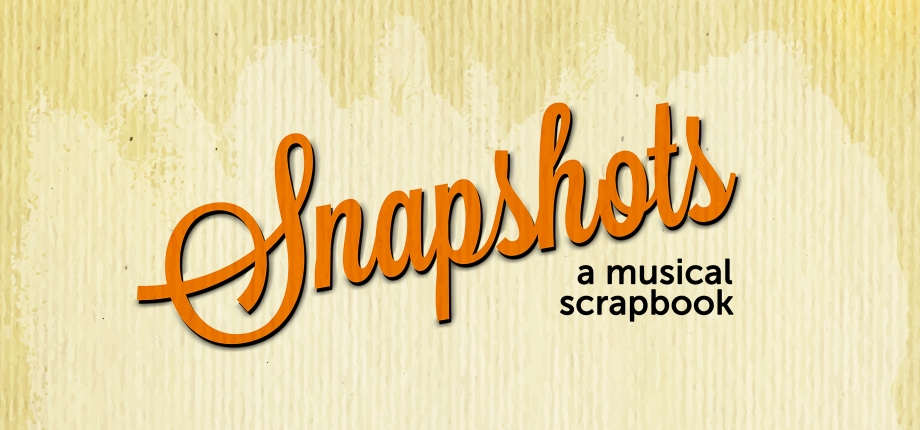The image appears to be designed as a promotional graphic, possibly a banner ad or part of a book cover, intended to advertise "Snapshots: A Musical Scrapbook." The central focus is on the title "Snapshots" written in a fun and feminine cursive font in pale orange. This title is prominently positioned in the middle of the image, tilting slightly. It has distinct black shadowing that adds depth to the text. Below "Snapshots," slightly off to the right, is the subtitle "A Musical Scrapbook" in a traditional black font. The background resembles stained, textured cardboard with a darker yellowish color along the edges and a lighter, smudgy section where the word "Snapshots" appears, creating an irregular yet appealing visual contrast that emphasizes the title. The image uses a muted color palette of yellows, oranges, tans, blacks, and whites, giving it a vintage, scrapbook-like aesthetic. Given its dimensions and design, it looks suitable for digital use, such as a Facebook banner or an e-book cover.